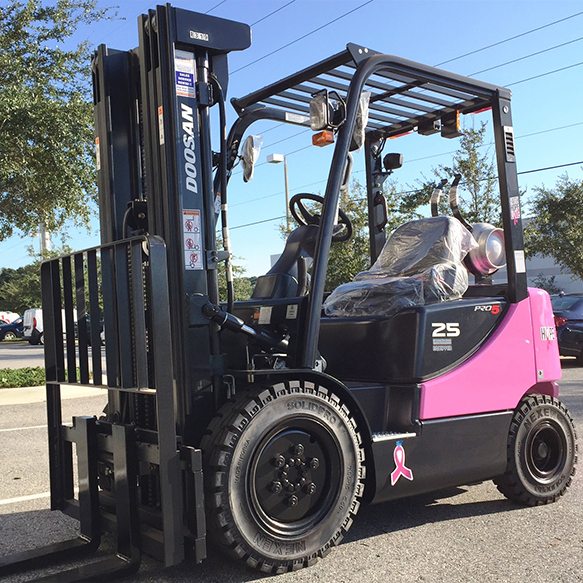The image features a close-up of a pink forklift, prominently displaying a breast cancer awareness ribbon. Positioned on the pavement outside, the forklift is centered in the frame with power lines and green trees visible in the background and blue sky above. The forklift's back wheel is smaller compared to the larger front wheel. 

The forklift includes various detailed components: on the right-hand side of its pink body is the breast cancer ribbon, and on the left is a vertical black section displaying "Dawson" along with some direction illustrations. The seat, located in the center, is covered with protective plastic as if brand new, with a steering wheel in front and the number 25 below. 

A headlight and possibly other lights or speakers are mounted on a grating above the seat, resembling a grill. In the background, the street pavement can be seen, along with parts of parked cars on both the left and right-hand sides of the image. 

The distinctiveness of the hot pink color likely sparks some discussion among drivers due to its uncommon appearance for such equipment.